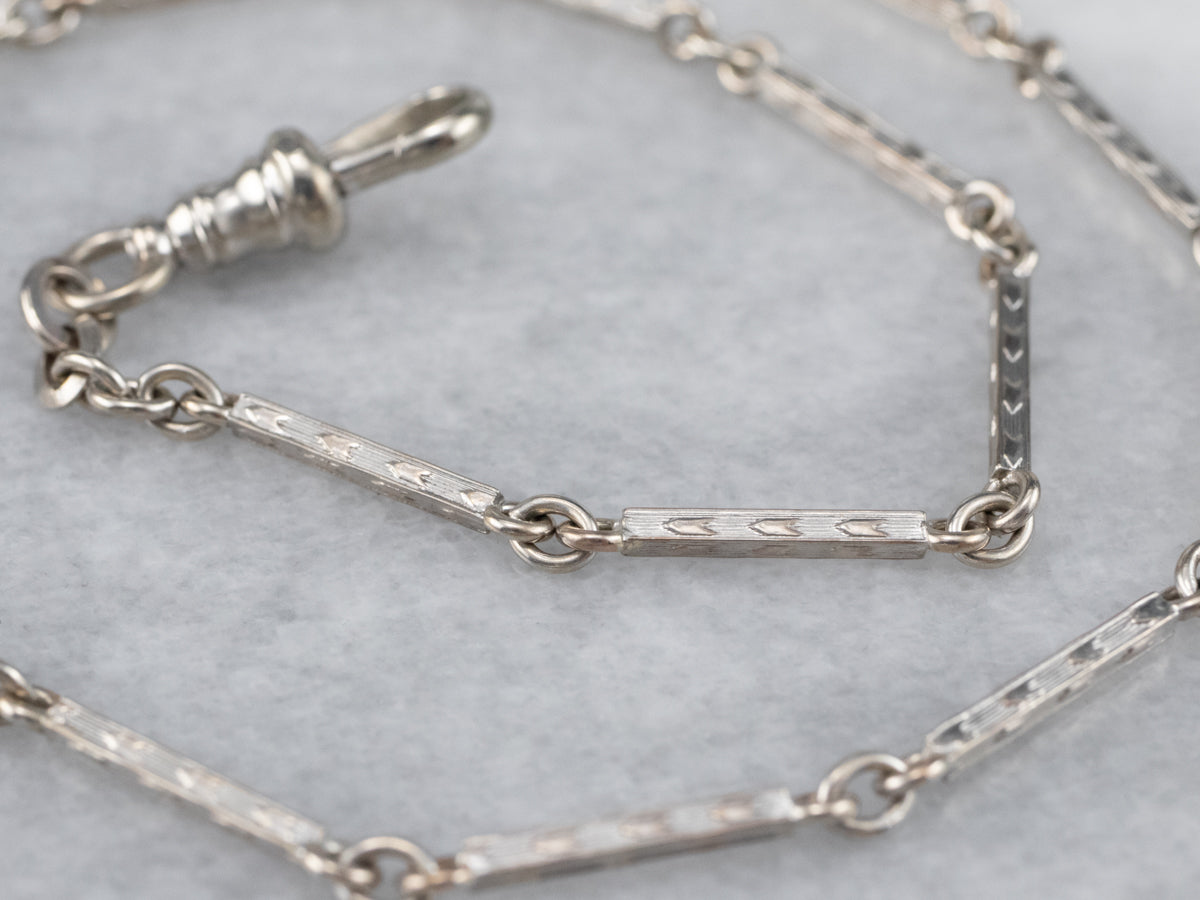The image depicts a highly polished, silver-colored necklace arranged in a coiled, spiral pattern on a flat surface, likely designed for fine jewelry display. The necklace is composed of individual solid bars connected by rings, with three small arrow-shaped designs etched into each section, giving it a distinct, intricate detail. The necklace's flexible construction suggests it would move easily when handled. Although not entirely visible, a beautiful clasp, resembling a lobster claw, is present at one end but lacks the connecting piece needed to secure it for wearing. The pristine condition of the necklace suggests it is well-maintained or possibly new.